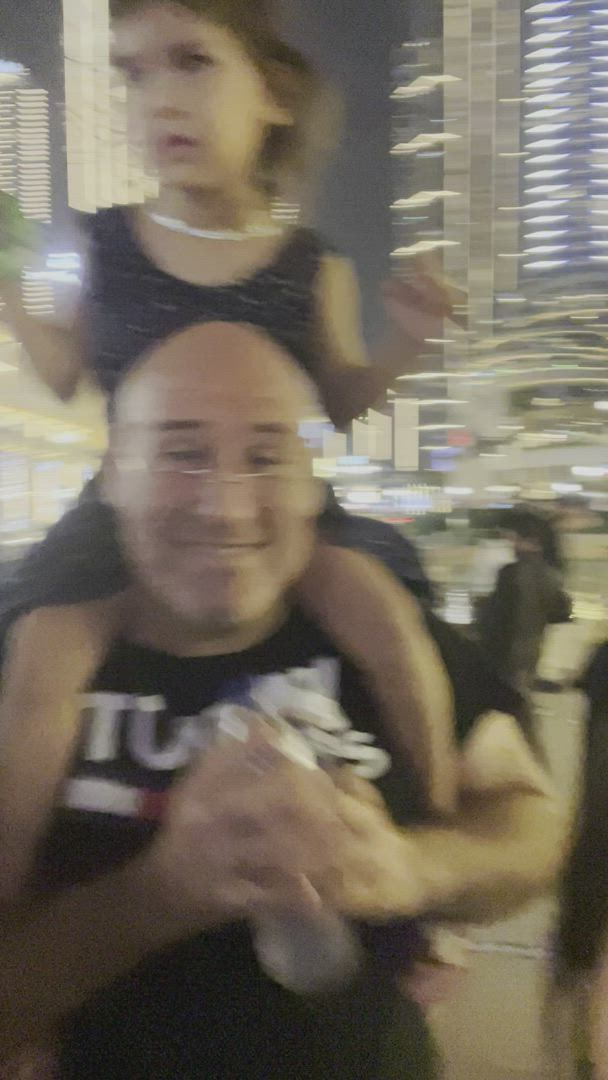In a blurry, out-of-focus photograph taken at night in a bustling urban setting with towering, illuminated skyscrapers, a bald man with glasses perched on his nose stands in the foreground, smiling directly at the camera. He is wearing a t-shirt with some white writing on it, partially visible with letters 'T' and a line under it. His hands are clasped in front of him, seemingly holding a water bottle. Sitting on his shoulders is a young girl, about three years old, with short brown hair. She wears a sleeveless, dark blue dress with white spots and a white necklace. Unlike the man, who looks into the camera, the girl gazes off to the side, her arms outstretched. The entire image is a blur of light and movement, encapsulating a fleeting moment in a vibrant cityscape.